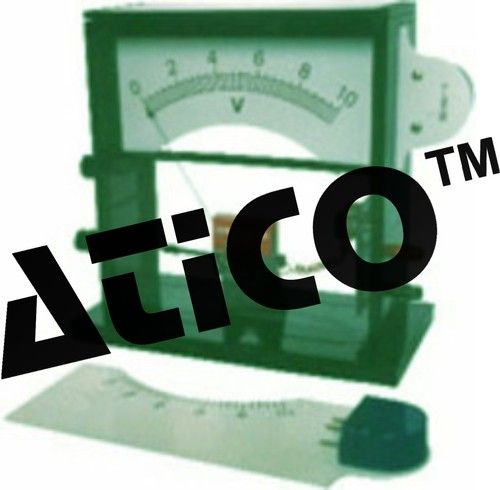The image features a meter with a distinct green metal frame resembling a window. At the top of the meter is a rectangular section displaying a semicircular scale marked with numbers from 0 to 10, including 2, 4, 6, and 8 sequentially, with 10 on the far right. In the middle, below the curve, there's a letter 'V'. The meter includes two rectangular legs standing on a green rectangular board positioned on the ground. In front of this meter is a similar white meter. Overlaid on the image are the bold stylized black letters "A-T-I-C-O", with a small "TM" appearing in the top right corner of the 'O'. The 'A' in "A-T-I-C-O" resembles an unclosed rectangle, contributing to its distinctive appearance.